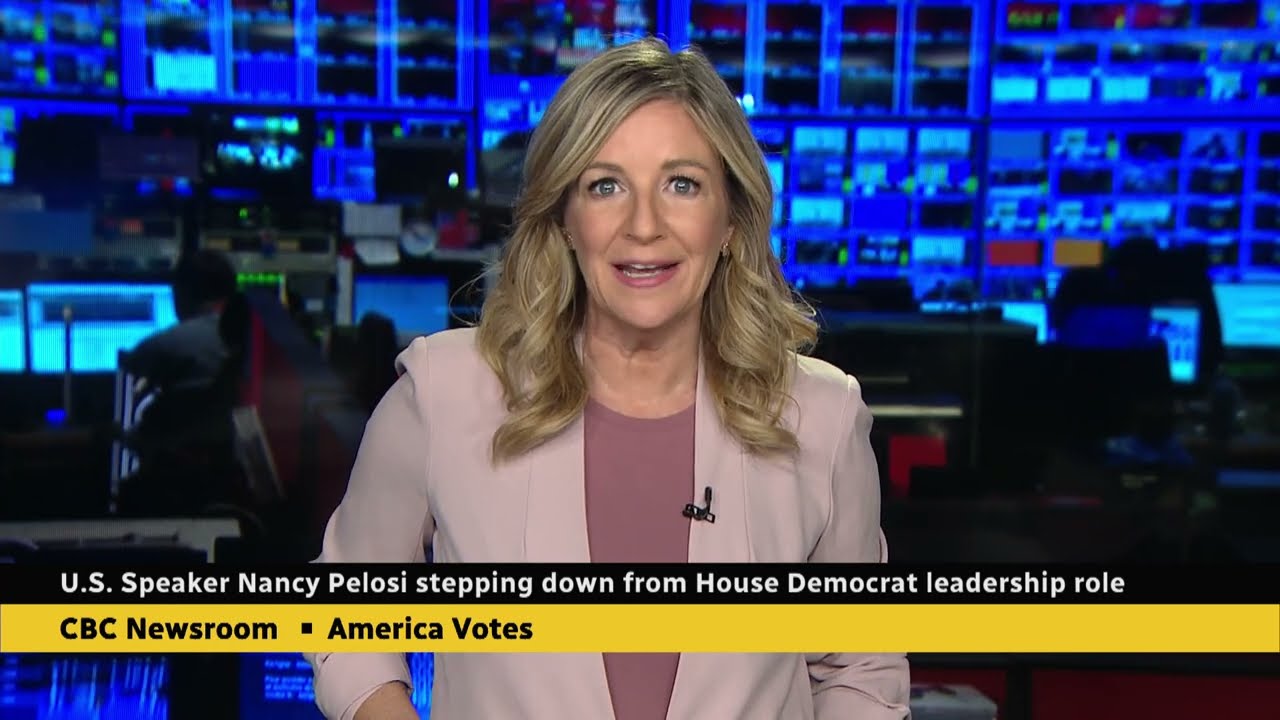In this detailed image, we see a news anchor at the center of a vibrant newsroom setting, presenting during what appears to be a live broadcast. The background is filled with a wall of multiple bright blue and black screens, displaying various video feeds. Several desks are visible with people working at them, though the details of these individuals are not prominent.

The central figure, a white woman with thin, slightly wavy blonde hair that falls just past her shoulders, is the focal point. Her hair is parted slightly off-center and curls gently at the front. She appears to be in the middle of speaking, her mouth open in mid-sentence, and her light green or blue eyes fixed on the camera.

She is dressed in a light pink blazer, under which she wears a mauve or light beige shirt. A small black microphone is clipped to the right lapel of her blazer, adding to the professional broadcast setup.

At the bottom of the image, a black banner with white text announces: "U.S. Speaker Nancy Pelosi stepping down from House Democrat leadership role." Directly below this, a yellow banner with black text reads: "CBC Newsroom America Votes." The setting of the image, combined with the detailed description of the anchor and the textual information, suggests a live coverage scenario within a bustling newsroom environment.